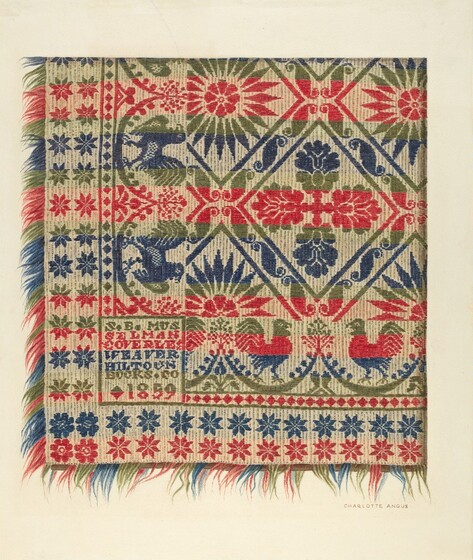The image depicts a highly detailed illustration resembling a traditional woven blanket. The blanket features an intricate and symmetrical pattern that includes a series of roosters, stars, flowers, and diamond shapes. The outer edge of the blanket is adorned with stars and flowers, transitioning inward to diamonds and then roosters. The inner section showcases an abstract pattern typical of traditional blanket designs. The primary color of the blanket is beige, complemented by multicolored details in blue, green, and red, which are also seen in the fringe along the edges. Woven into the fabric at a corner, the text reads: "S.B. Musselman Coverlet Weaver Hilton Books Company 1859." This suggestion of words and date indicates the company and year of creation, emphasizing the cultural and historical significance of the blanket.